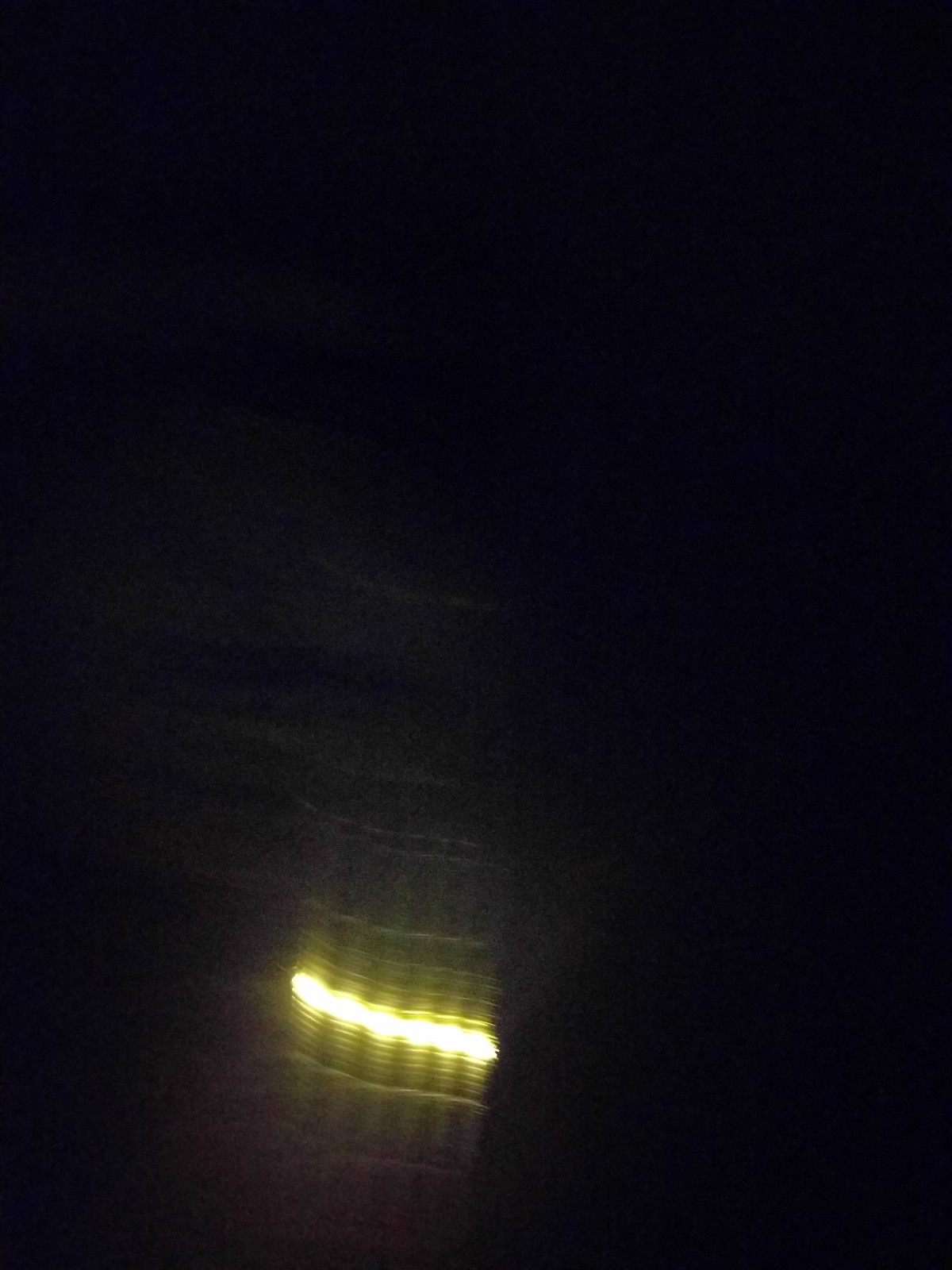The image features a predominantly dark, tall rectangle. Near the bottom left of the rectangle, there's a notable grouping of six bright yellow orbs. These orbs appear to be lights, possibly from a vehicle such as a bicycle or a motorcycle, as a blurred, indistinguishable object resembling a license plate can be seen below them. Above and below the lights, there are streaks of blur that create linear patterns, adding to the obscurity of the scene. The overall lack of clarity in the image makes it challenging to definitively identify the objects within it.